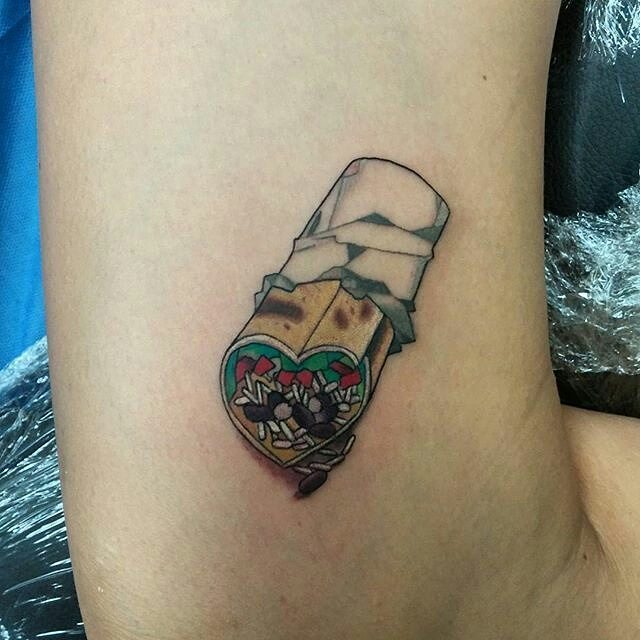The image depicts a tattoo located on the forearm of an individual with a light to olive skin tone, possibly indicating a Mediterranean or Hispanic background. The tattoo itself is an intricate and whimsical design, featuring a heart-shaped burrito. Within the heart-shaped tortilla, colorful elements such as beans, rice, lettuce, and tomato are meticulously detailed. The burrito's base is wrapped in a crinkled wrapper, adding to the realism and playful nature of the artwork. In the background, the headrest of a car is visible, tightly wrapped in black leather and encased in plastic wrap. Additionally, a piece of blue cloth is noticeable behind the arm, contributing to the vibrant and textured composition of the scene.